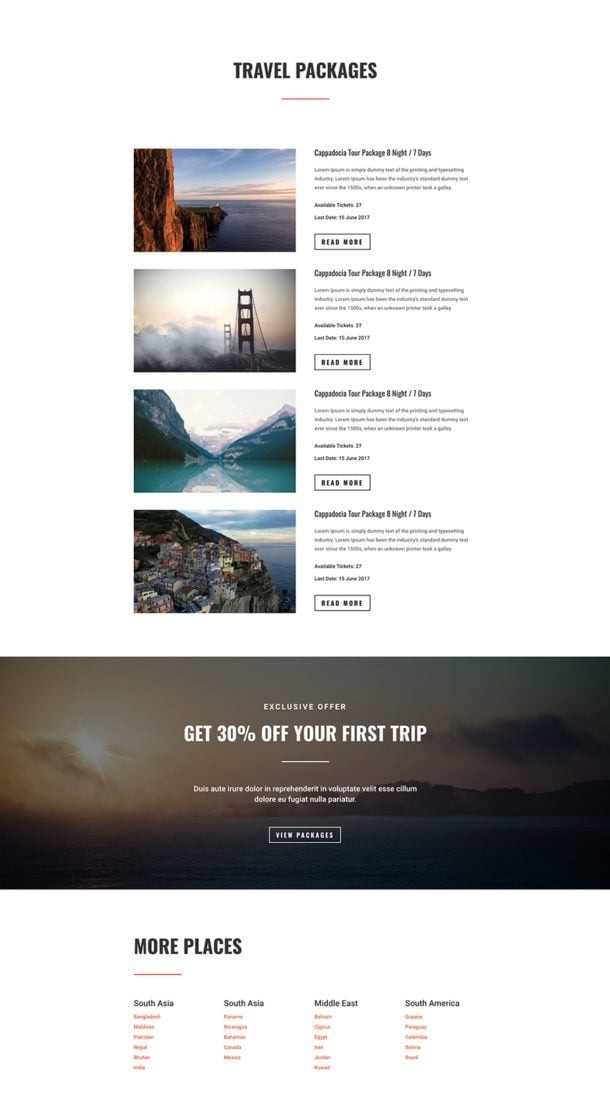The image showcases a website offering four distinct travel packages, each accompanied by a small image on the left that illustrates the destination. The first image depicts a picturesque mountainous terrain with the sea stretching below. The second image captures an iconic red bridge set against a clear sky. The third shows a stunning blue lagoon flanked by rocky formations. The fourth features a charming village perched on cliff edges, overlooking the shore.

Each travel package provides information on the duration of the stay, detailing the number of nights and days included. The descriptions are succinct and written in small text, making it difficult to read the specifics without clicking on the "Read More" button available next to each package for expanded details.

Beneath these packages, a prominent rectangular banner announces an exclusive offer in large text: "Get 30% Off Your First Trip." Below this message is a "View Packages" button. Further down, another section invites users to explore additional destinations with headings such as South Asia, Middle East, South America, and others, offering a wide array of travel options to peruse.